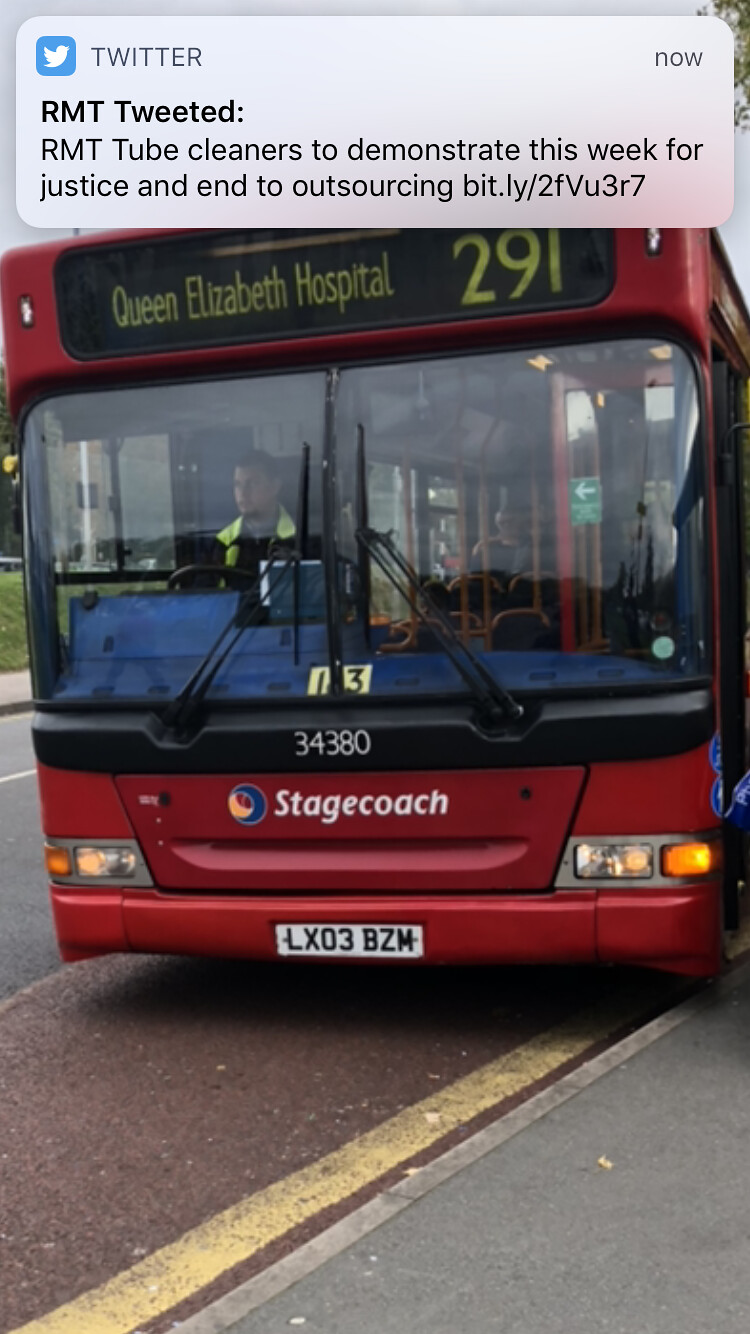The image captures a red bus, prominently displaying the word "Stagecoach" in white on its front bumper. The bus is positioned partially on a sidewalk, potentially picking up or dropping off passengers. The bus has a European-style license plate with the black text "LX03 BZM" on a white background. Above its expansive windshield and visible windshield wipers, the destination signage reads "Queen Elizabeth Hospital 291" in yellow on black. On the bus, the driver is seen on the right side, indicative of a left-hand driving country. Overlaying the image, a Twitter notification is visible at the top, featuring the Twitter logo and text, "RMT tweeted: RMT tube cleaners to demonstrate this week for justice and end to outsourcing," followed by a shortened URL link.